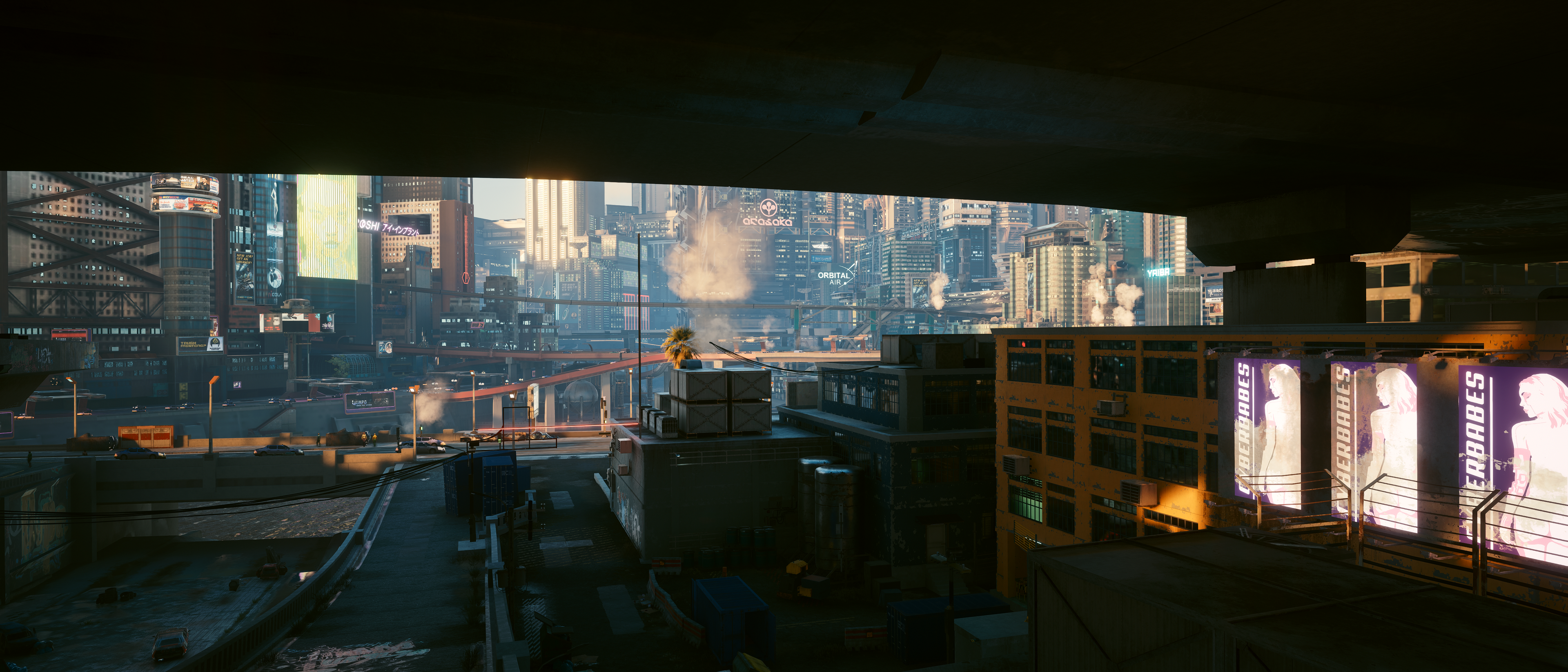This image captures a detailed cityscape as viewed from underneath a vast highway overpass, creating a striking juxtaposition between industrial elements and urban grandeur. The photograph, which appears to be in color and possibly computer-generated due to its overly manicured appearance and somewhat unnatural smoke, is taken in landscape format. From the vantage point beneath the overpass, which has two sturdy pylons visible on the right, the foreground reveals buildings shrouded in shadow but interspersed with illuminated signs. To the left is an orange building suggestive of a warehouse or factory, aligning with the industrial aesthetic underscored by train tracks and a visible train car below. In the distance, the scene opens up to a sprawling cityscape dominated by towering skyscrapers, their tops cut off by the overpass's roof, further adding to the perspective's dramatic effect. The urban tableau is populated with details like steam and scaffolding, evoking the energy and complexity characteristic of a large metropolitan area.